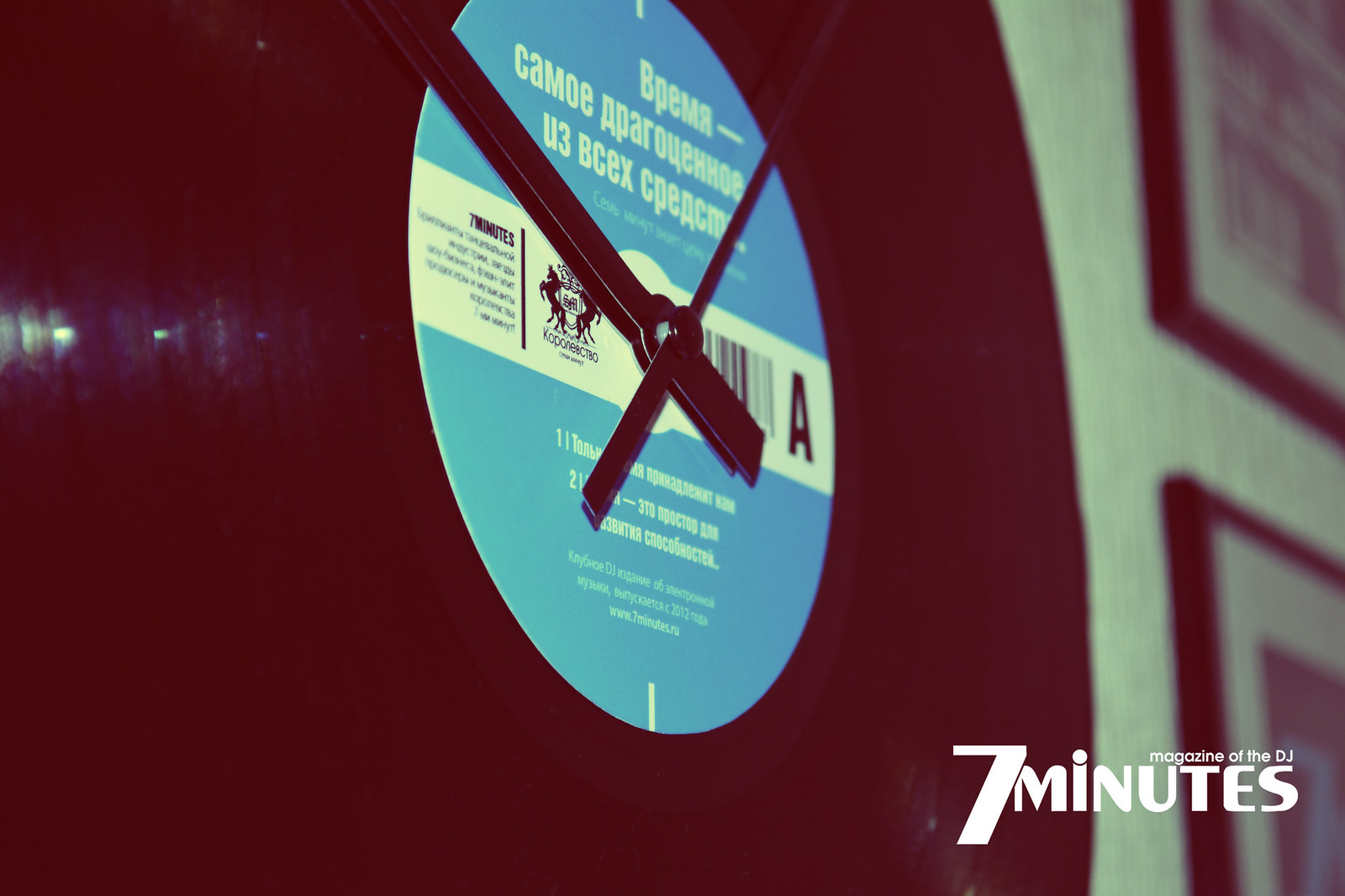The image features a clock cleverly crafted from a vinyl record, prominently displaying a blue label written in a foreign language with an indistinct capital black "A." The record, acting as the clock face, includes distinct hour and minute hands. Notably, the bottom right-hand corner of the image bears the inscription "seven minutes" in large white letters, followed by "magazine of the DJ" in smaller white text. The clock is mounted on a textured wall resembling wallpaper, characterized by subtle lines. The background includes other black-framed, black-and-white photographs, although they appear out of focus.